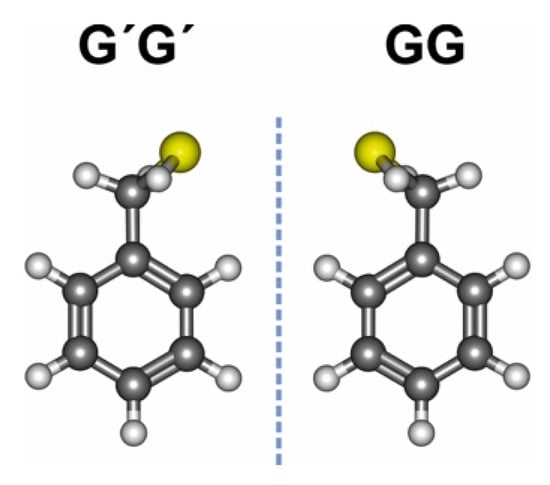The image is a color drawing of two molecular structures separated by a blue dashed line down the middle. On the left side, the structure is labeled "G" in black text, while on the right side, it is labeled "GG." Both structures resemble DNA molecules with eight white ends connected by seven black segments in between. The structures appear to be mirror images of each other. Each main molecule forms a somewhat circular shape with ends extending outward. Notably, on the right side, a yellow ball is attached to one of the black ends, positioned on the opposite side compared to its counterpart on the left. The intricate hexagonal arrangement of the primary molecules is predominantly gray with white centers, and the smaller white molecules are simply white without additional coloration.